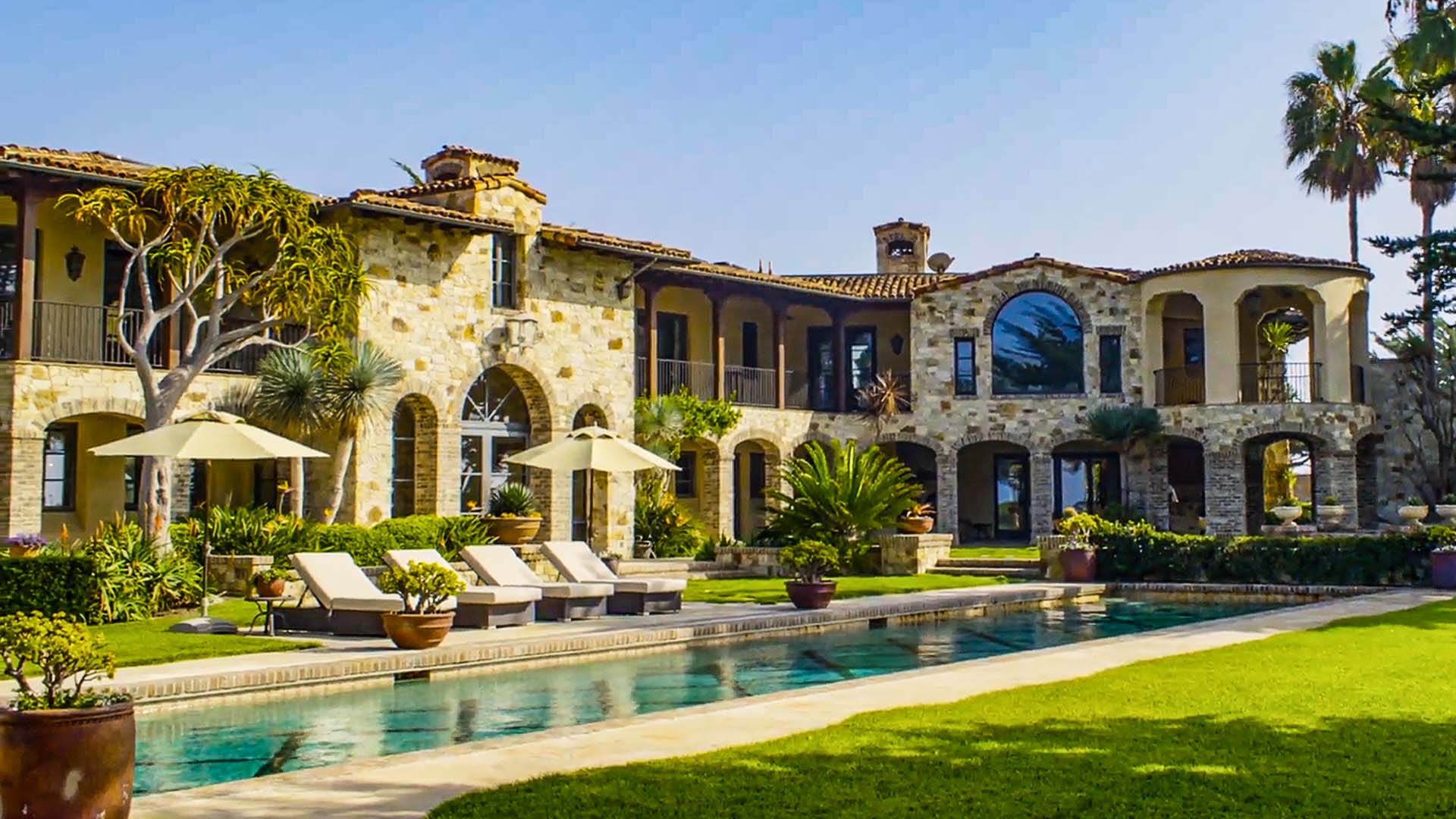This image captures a picturesque backyard of a mansion, showcasing a splendid blend of architecture and landscaping under a clear blue sky. The mansion is constructed with tan bricks and features distinctive terracotta-tiled roofs. The house dominates the background, stretching almost the entire length of the image, and exhibits elegant stone archways and large glass windows, alongside a noticeable second-level patio with numerous doors. An expansive, rectangular pool, nearly the same length as the mansion, graces the foreground, reflecting the blue of the sky. Surrounding the pool is a lush, green lawn interspersed with various tropical plants and decorative vases. On the left side of the pool, four identical cushioned lounge chairs are stationed, flanked by two beige umbrellas. Tall palm trees are visible on the right, their shadows cast on the verdant lawn. In the bottom left, a conspicuous vase with a tiny plant adds to the charm of the tastefully landscaped environment.